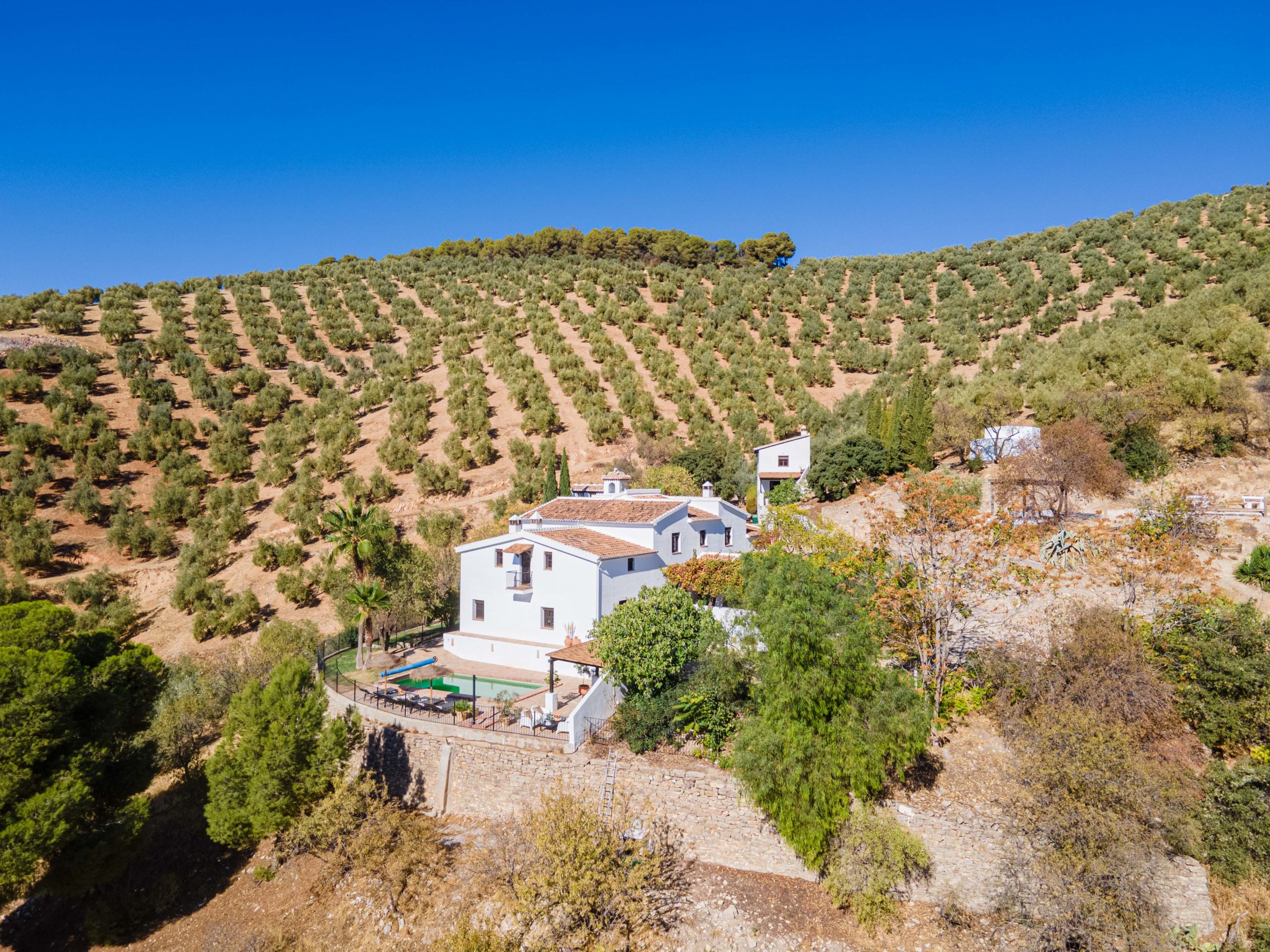The image showcases an aerial or drone view of a picturesque countryside landscape with a prominent, older-looking, large white home at its center. The house, which is multiple stories tall, features a light brown roof that complements the surrounding brown dirt. In front of the home, a spacious swimming pool is visible, accompanied by pool chairs and a patio area. The property is surrounded by a lush array of greenery, including several palm trees on the left and bushes to the right, all supported by a sturdy stone retaining wall beneath the home. Adjacent to the right of the main house stands a tall structure resembling a treehouse. The background reveals rolling hills with meticulously lined green shrubs, suggesting an agricultural setting. The sky above is a striking, almost artificial-looking bright blue, adding a vivid contrast to the earth tones below. The overall palette of the image includes green, light blue, dark blue, gray, black, and white, with no text present in the photo.